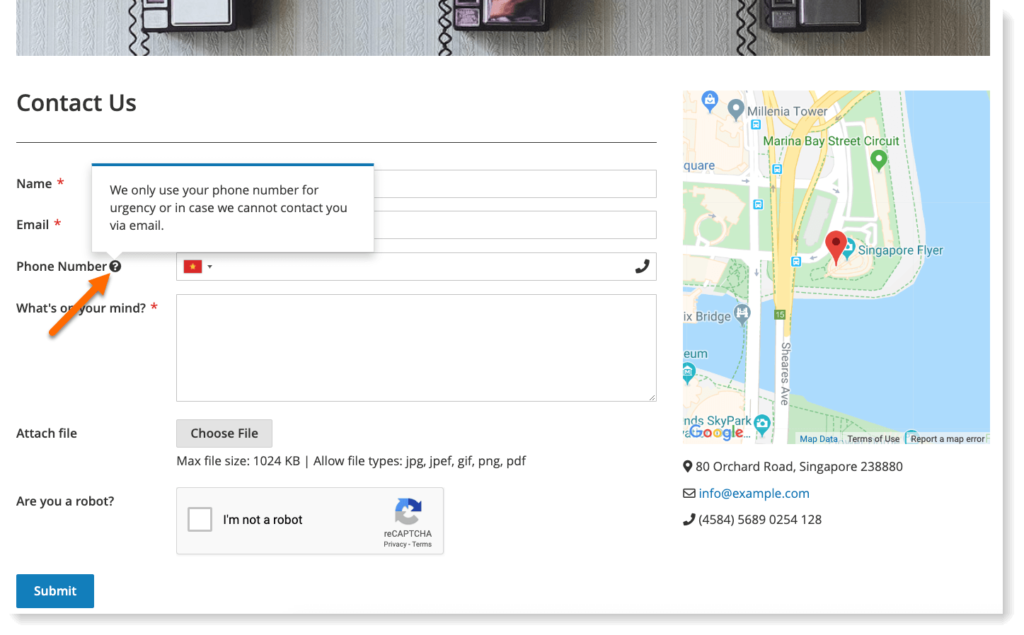This image is taken from a website's "Contact Us" page. At the top, an illustrative banner displays vintage telephones with long cords, evoking a sense of nostalgia. Below this, there is a form where users can enter their name, email, and phone number. A question mark icon next to the phone number field has been clicked, revealing a tooltip that explains the phone number will only be used in urgent situations or if email contact fails.

The phone number field is highlighted by a red button to its right. Beneath the form, a black telephone icon is situated next to the text "What's on your mind?" prompting users to leave a message in a text box. There is also an option to attach a file using a "Choose File" button, along with a note specifying the maximum file size allowed.

Towards the bottom of the page, there is a reCAPTCHA widget with the label "I'm not a robot" for spam prevention, and a "Submit" button located at the far left-hand bottom corner. To the right of the contact form, a map shows the location of the business. At the very bottom, the company's address, email, and phone number are listed for additional contact options.